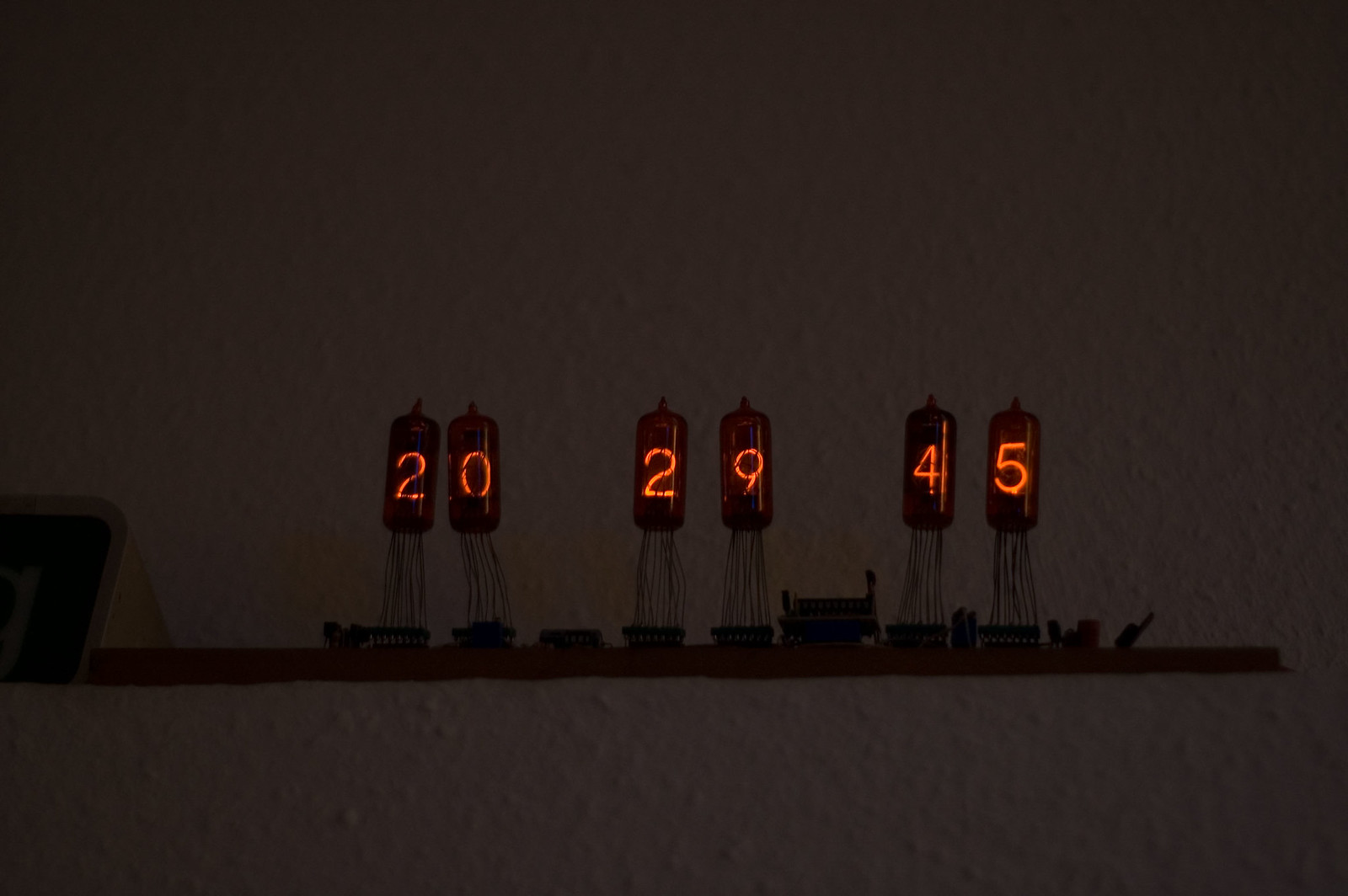The image features a digitally generated side view of a circuit board set against a dark, textured background. The board supports six cylindrical components arranged in pairs, each emitting orange neon signage displaying the numbers 20, 29, and 45 from left to right. These components are elevated above the board by thin wires or poles. On the left side of the board, there's a larger vertical rectangular structure, while a smaller rectangular piece is situated between the components labeled 29 and 45. The overall scene is presented with a dark grey or black backdrop, highlighting the illuminated numbers and the intricate circuitry.